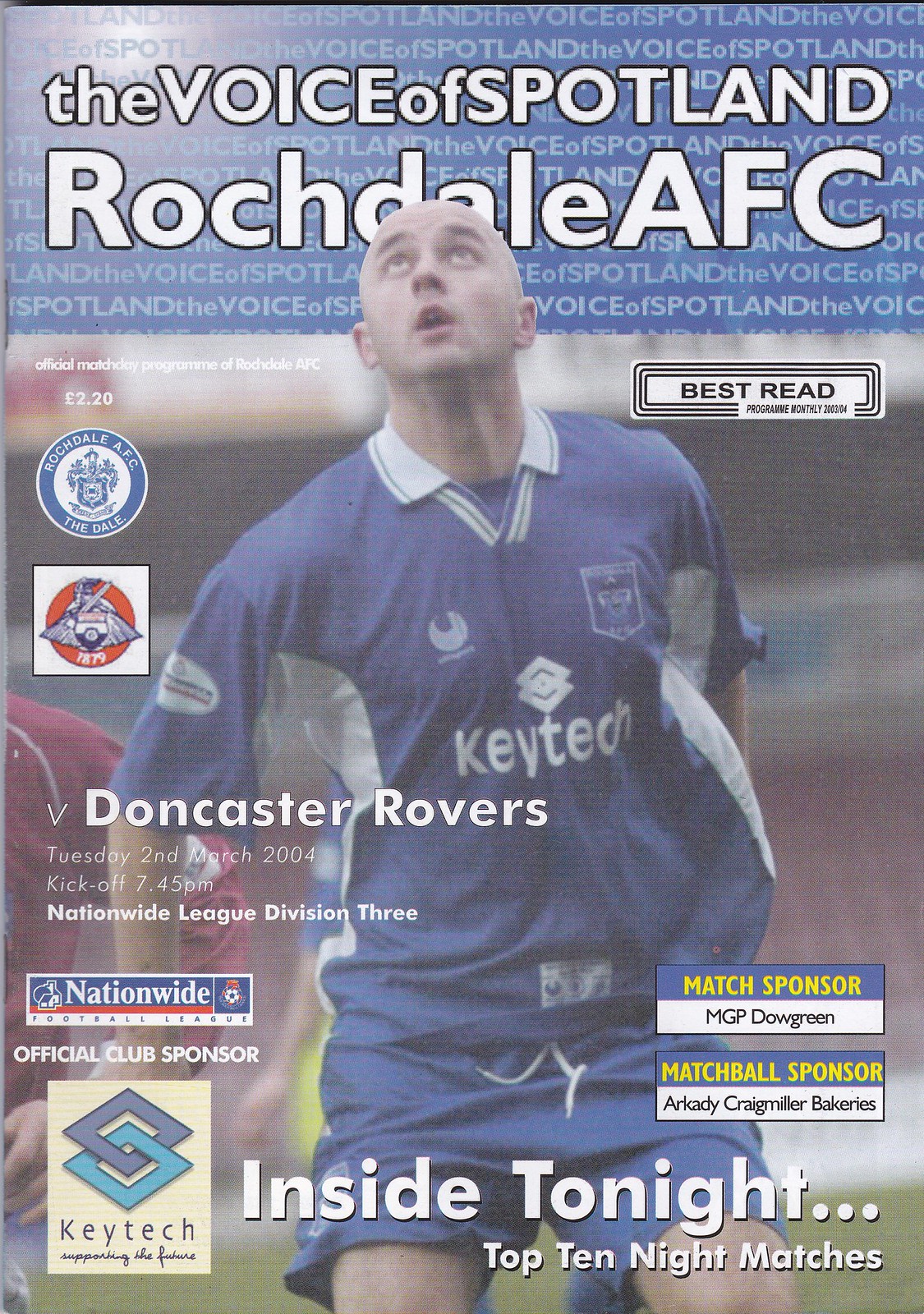The magazine cover features "The Voice of Spotland, Rochdale AFC" prominently displayed at the top against a vibrant blue backdrop with repeated lines of the same phrase. Below this banner, on the left-hand side, it states, "Official Match Day Program of Rochdale AFC" with the price listed as £2.20. The central image is of a soccer player in a blue collared shirt emblazoned with "Key Tech" and matching blue shorts, looking up towards the sky.

Further down the cover on the left side, a blue and white circular logo reads "Rochdale AFC, The Dale." Just beneath this logo is the match information: "Doncaster Rovers, Tuesday, 2nd March 2004, kickoff 7.45 PM, Nationwide League Division III." Adjacent to this, there is the Nationwide Football League logo followed by the text "Official Club Sponsors."

In the bottom left corner is a cream-colored rectangle featuring a logo of two intertwined diamonds and the text "Key Tech, supporting the future." Just to the right of this, in larger letters, it reads: "Inside Tonight... Top Ten Matches." Above this section, sponsor details are presented in a two-tone blue and white rectangle: "Match Sponsor: MGP Dow Green" in yellow and black text, and an identical rectangle below that notes "Match Ball Sponsor: RKD Craig Miller Bakeries."

On the right side, under the main blue banner, is a logo within a white rectangle lined with three black borders and the words "Best Read." The cover is detailed and visually organized to highlight key match and sponsor information, drawing the viewer's attention to the excitement of the event.